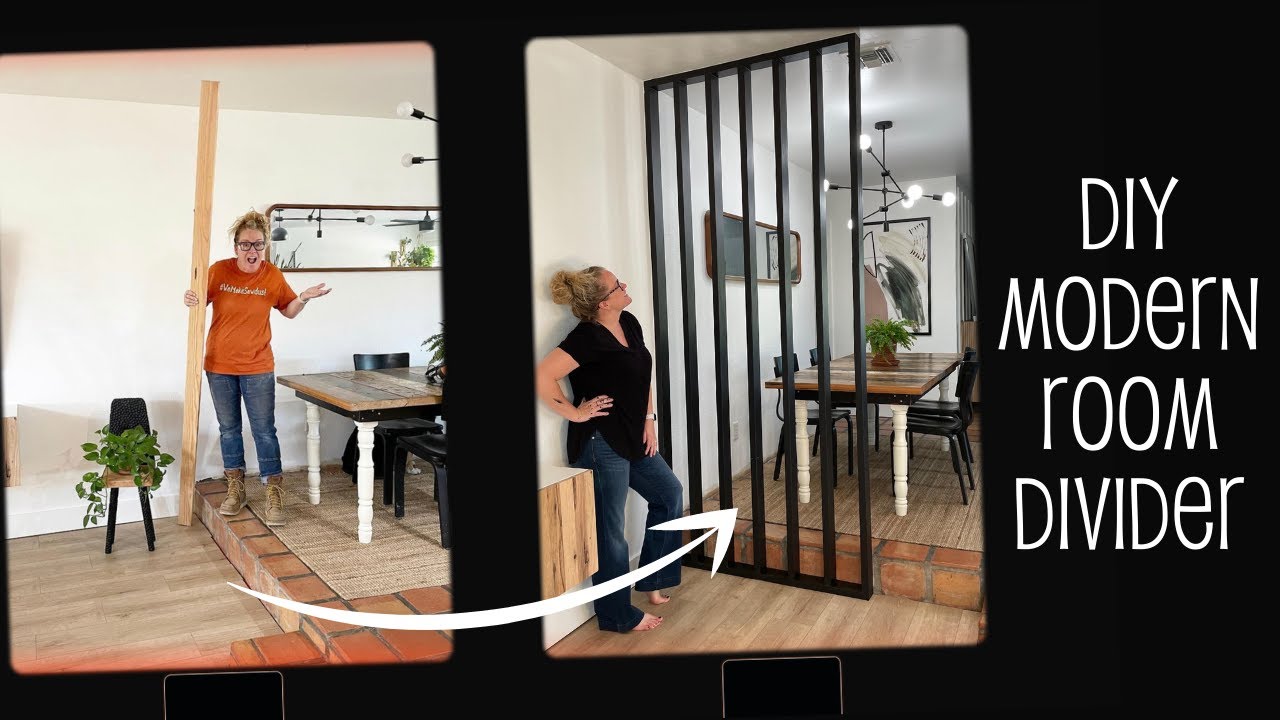The composite photographic image features a DIY modern room divider project with white text on a black border reading "DIY Modern Room Divider." On the left panel, a white woman wearing an orange t-shirt, blue jeans, and brown boots is standing on a brick platform. She holds a plank of wood with one hand while her other hand is raised in exasperation, her mouth open, and glasses perched on her face. A black-seated chair with a green plant sits nearby, and behind her, a wooden table, a mirror reflecting a ceiling fan, a frame, a white wall, and a hardwood floor complete the room. An arrow points to the right panel, depicting the same woman now in a black t-shirt, blue jeans, and barefoot, standing on the floor with one hand on her hip. She looks proudly at a newly constructed room divider made of wood. Through the divider, a dining room is visible with a table, four chairs, a painting, an overhead chandelier, and a mirror on the back wall. The image effectively captures the transformation and accomplishment from start to finish.